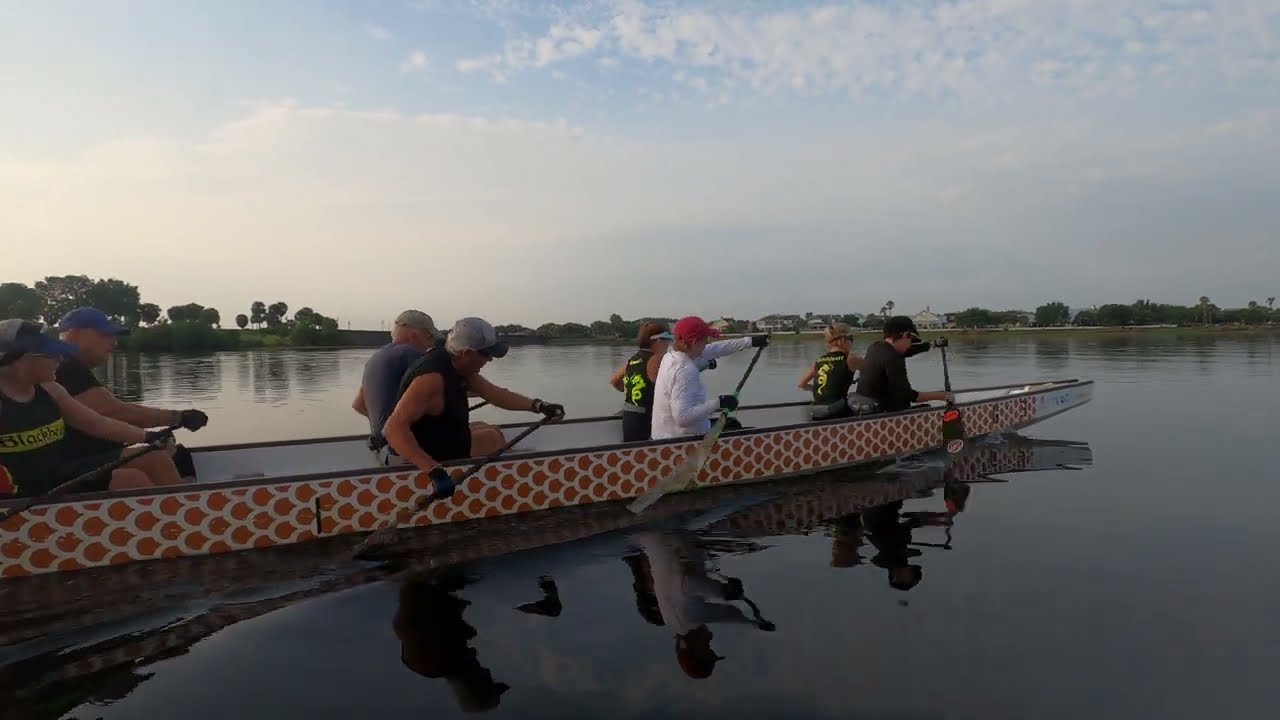In a scenic setting with a light blue sky dotted with patchy white clouds, a group of eight mature adults, consisting of both men and women, are rowing seamlessly in a white boat with an orange scale-like pattern. The water beneath them is dark, and the lush backdrop features green vegetation, towering mountains, and scattered trees, giving the impression that they are on a serene lake or possibly a river. The rowers, dressed in a mix of long sleeves, tank tops, and wearing hats or visors, are concentrated on their paddling, causing little disturbance to the water's surface. The distant shores host various islands and houses with gray roofs, adding to the picturesque landscape. Although not a professional photograph, it effectively captures the essence of a dedicated rowing team amidst nature’s splendor.